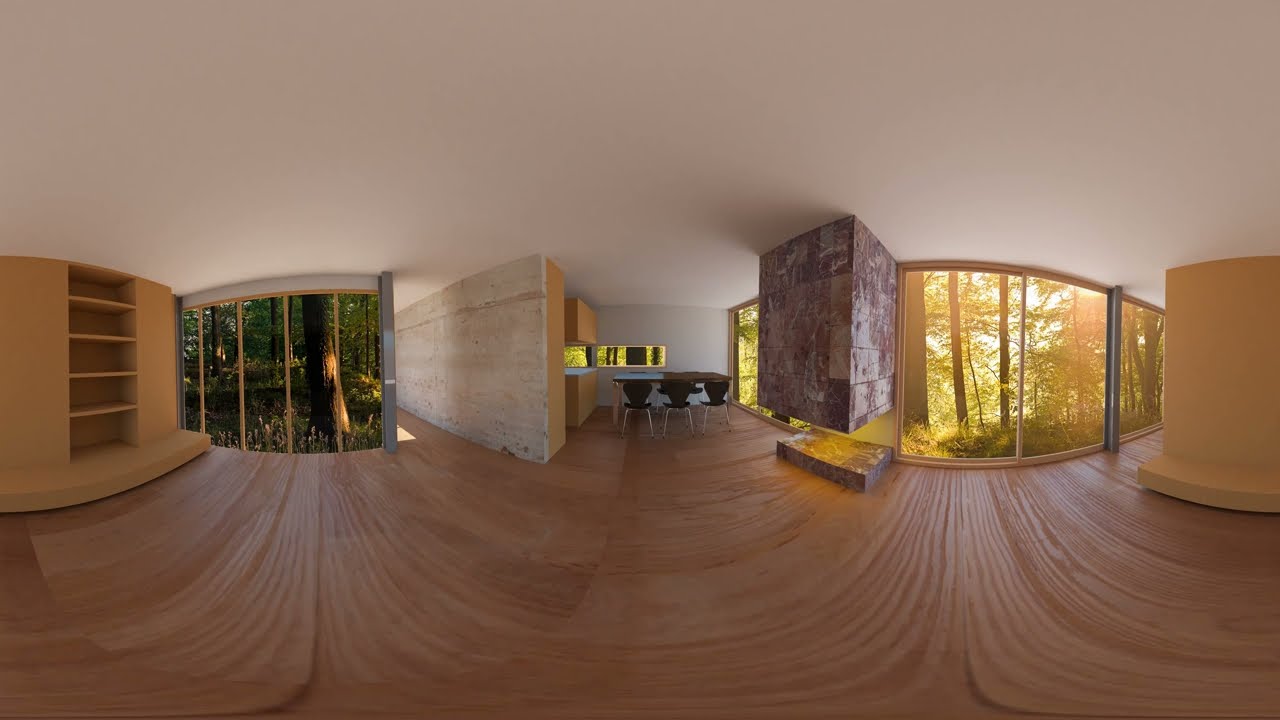This image reveals a cozy room taken with a 360-degree lens, lending a fisheye effect to the scene. The room has a rich wooden floor with prominent grain patterns that curve and swirl due to the lens distortion. The ceiling is an immaculate white, while the walls are a mix of white and wood-colored tones. On the left side, there is a built-in brown shelf unit, adding functional decor to the space. Towards the right of the center is an abstract, possibly non-functional fireplace. The room is flooded with natural light from floor-to-ceiling glass walls, offering a stunning view of a verdant forest outside, with sunlight filtering through the trees. In the middle of the room, there is a table surrounded by multiple chairs featuring metal legs and black backs. This serene, sunlit room gives the impression of a treehouse nestled amidst lush greenery.